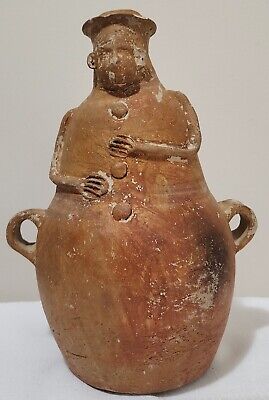The photograph captures an ancient artifact that appears to be an old, scuffed-up vase or jug. The object, seemingly made of baked clay, exhibits tones of brown and dark orangish-red, with areas showing wear and small flecks where the finish has worn off, giving it a distinctly aged look. The vase is pear-shaped, resembling a snowman structure, with two small, thick round handles on either side. These handles are designed for picking the item up, possibly placing thumbs or forefingers through them.

The central figure carved into the vase features a person's face, though the details are quite faded. The head of the figure is topped with a hat that forms part of the vase's upper section. The figure's arms wrap around its chest and mid-waist, with fingers extended, visible around the body. Running down the front of the figure's chest are four buttons, though they might number three, as the fourth could be obscured by the hands. The background of the photo is accented with a teal top and white bottom, emphasizing the strikingly designed object that occupies about 80% of the image frame.